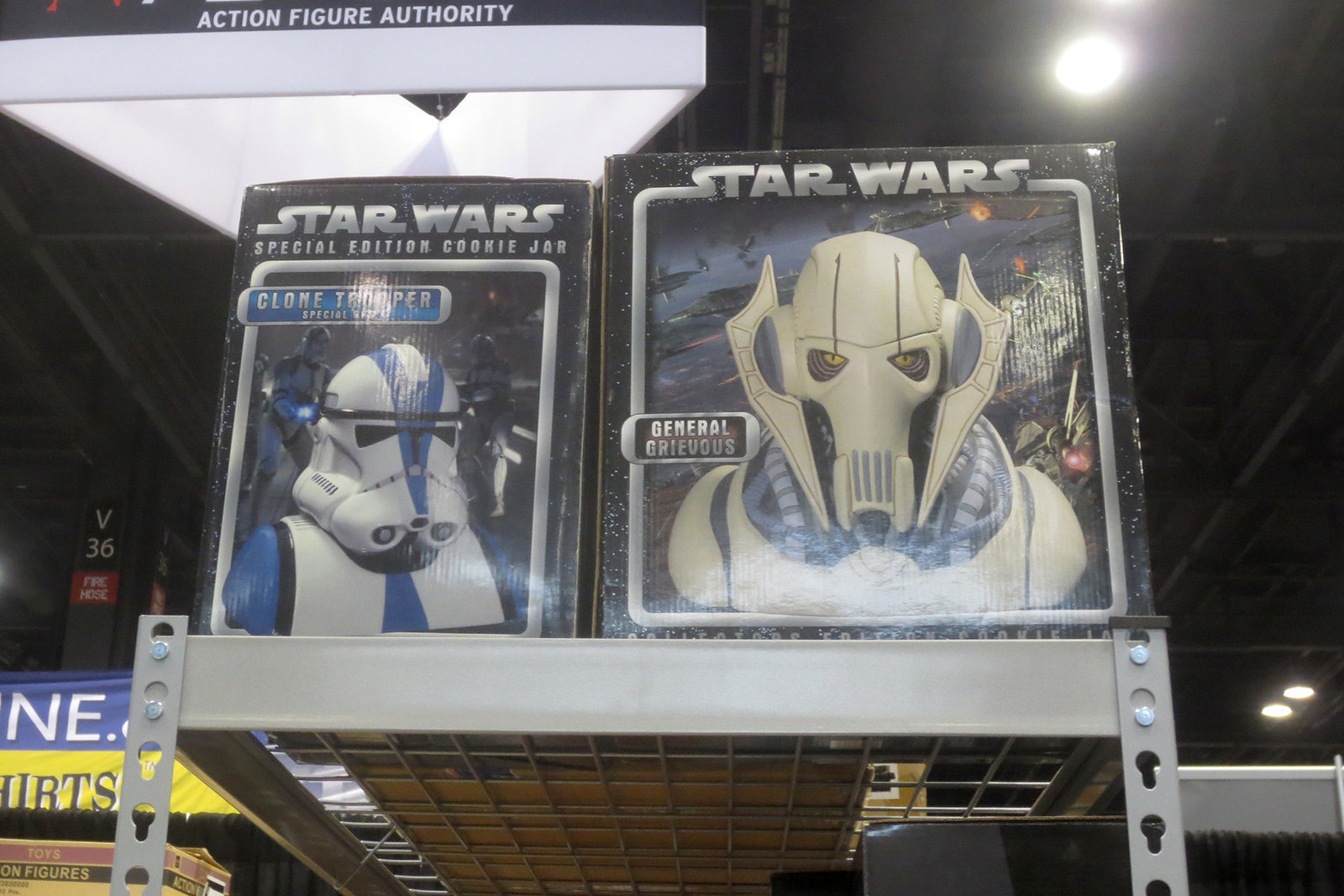The image captures a segment of a store environment, possibly a collectible sale or a Comic Con event, featuring Star Wars memorabilia prominently displayed on metal shelving. At the top left, a sign reads "Action Figure Authority" in white text against a black background, providing a hint of the setting's specialty. Center stage are two boxed items, both positioned directly in the middle of the image. The left box displays a "Star Wars Special Edition Cookie Jar" depicting a Clone Trooper with blue accents on his armor, while the right box showcases a figure of General Grievous with his distinctive skeletal appearance, complete with yellow eyes and tubing around his neck. The shelves are a gray metal, and the background includes ceiling lights, reinforcing the indoor setting. The colors in the image span blue, yellow, white, red, gray, pink, and black, further enhancing the vivid display of this vintage toys collection.